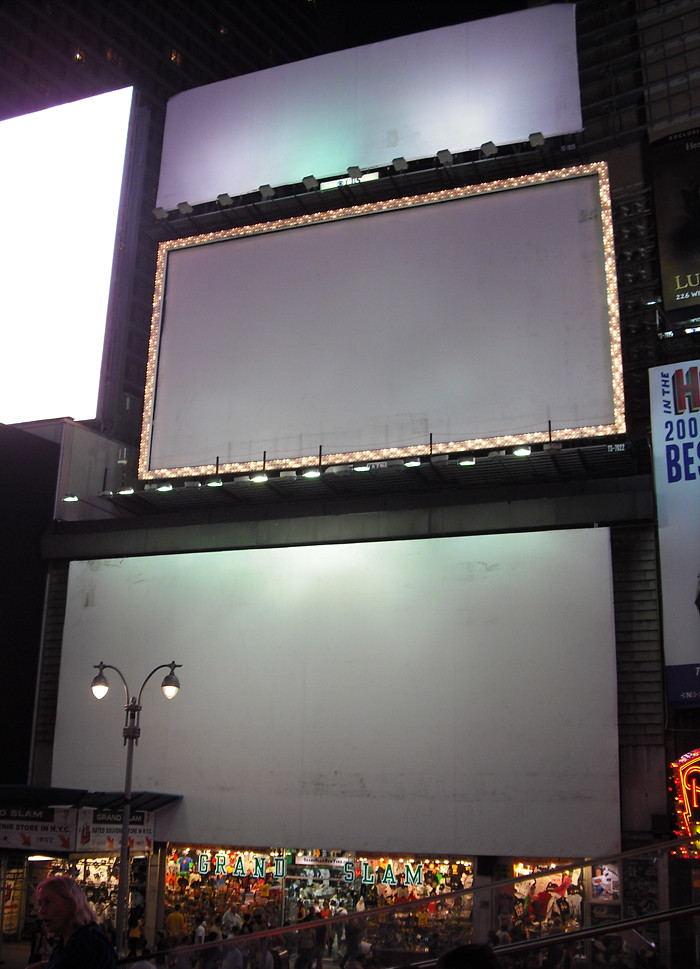The photograph captures a bustling yet somewhat tranquil nighttime city street, exuding a sense of urban elegance. In the foreground, there is a storefront emblazoned with the name "Grand Slam" on its window. The store radiates with vibrant colors from within, though the window does not reveal specific details of the interior. A few pedestrians are discernible on the sidewalk in front of the store, adding life to the scene.

Prominent in the upper part of the photograph are three large, blank screens which dominate the urban landscape. The first screen, situated to the far left, is of a grayish hue. Beneath this screen stands a distinctive lamppost, characterized by its V-shaped design that splits and gently curves downwards, each arm supporting a glowing white bulb.

Above this is another sizeable rectangular screen, bordered with golden yellow lights forming a gilded frame that adds a touch of opulence. The third screen, positioned slightly higher, is similarly grayish but is distinguished by a few brighter white lights along its lower edge.

To the left of the frame, there's a glimpse of yet another screen, strikingly bright white, though only partially visible. Despite their imposing presence, all the screens remain unlit, offering no images or advertisements, which adds a peculiar yet serene quality to the nighttime city street atmosphere.